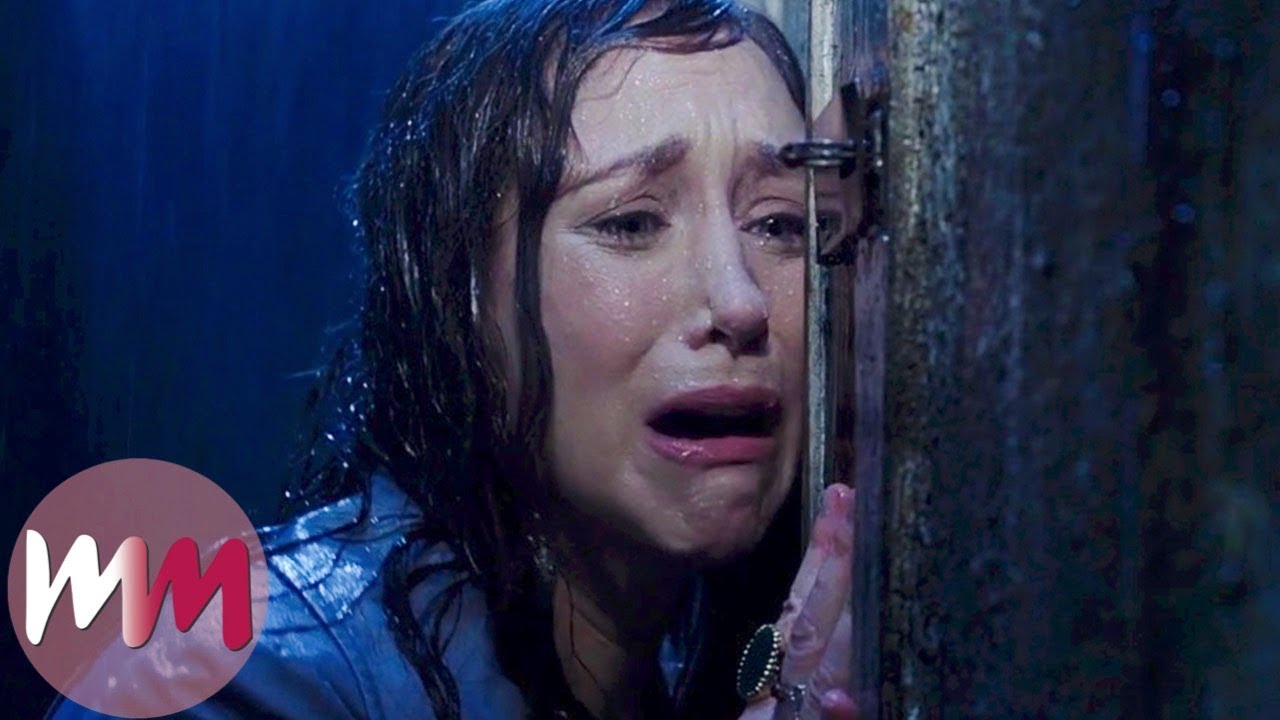This image captures an intense scene from an unidentified 80s or 90s movie. The distraught woman, drenched from the rain, presses her face and hand— which sports a prominent oval-shaped ring—against a weathered brown stone wall or door. Her light blue rain jacket is soaked, emphasizing her distress and the heavy rainfall. The colors in the scene are dominated by deep blues, blacks, grays, and touches of pink, alongside the natural flesh tones. Adding to the scene's complexity, a circular overlay with the letters "MM" transitions in color from white to dark pink, positioned in the bottom-left corner. The woman's expression of fear or sorrow, coupled with the surrounding elements, conveys a sense of urgency and helplessness as she seems to be either trapped outside or desperate to escape the rain and her predicament.